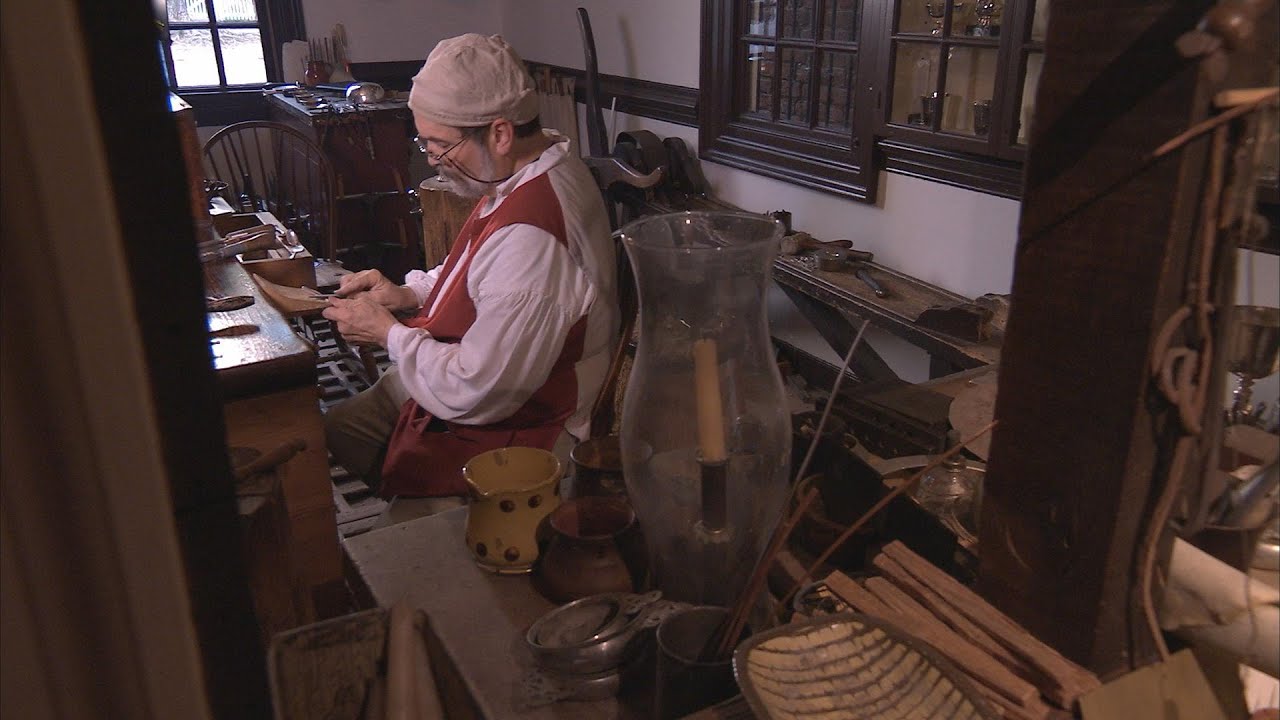In this photographic image, an older man sits centrally in a well-organized, indoor workshop. He wears a brown knit stocking cap and wire-rimmed glasses with eyeglass holders, paired with a red vest over a white, billowy shirt. The man, distinguished by his whiter beard, appears deeply focused on whittling a piece of wood. 

He is seated on a bench in front of a wooden table cluttered with tools and materials, including bowls, jars, and dishes. The backdrop showcases a setting reminiscent of an old-fashioned workshop or perhaps a recreated pioneer village. The room features white walls with dark wooden paneling and is adorned with various antique tools, rusty iron implements, and old-fashioned clay cups and mugs scattered on surfaces.

In the bottom right of the image, a box filled with assortments like sticks, a glass lamp, and a candle holder with a candle are visible. A post, running vertically, anchors the scene. The back wall, dominated by a large, dark wood panel window, suggests a cloudy day outside. Additional details include a smaller four-pane window frame in the top left corner, with a wooden chair and a table below holding more items. There is no text in the image, allowing the detailed setting and the man's absorbed activity to tell a vivid, historical story.